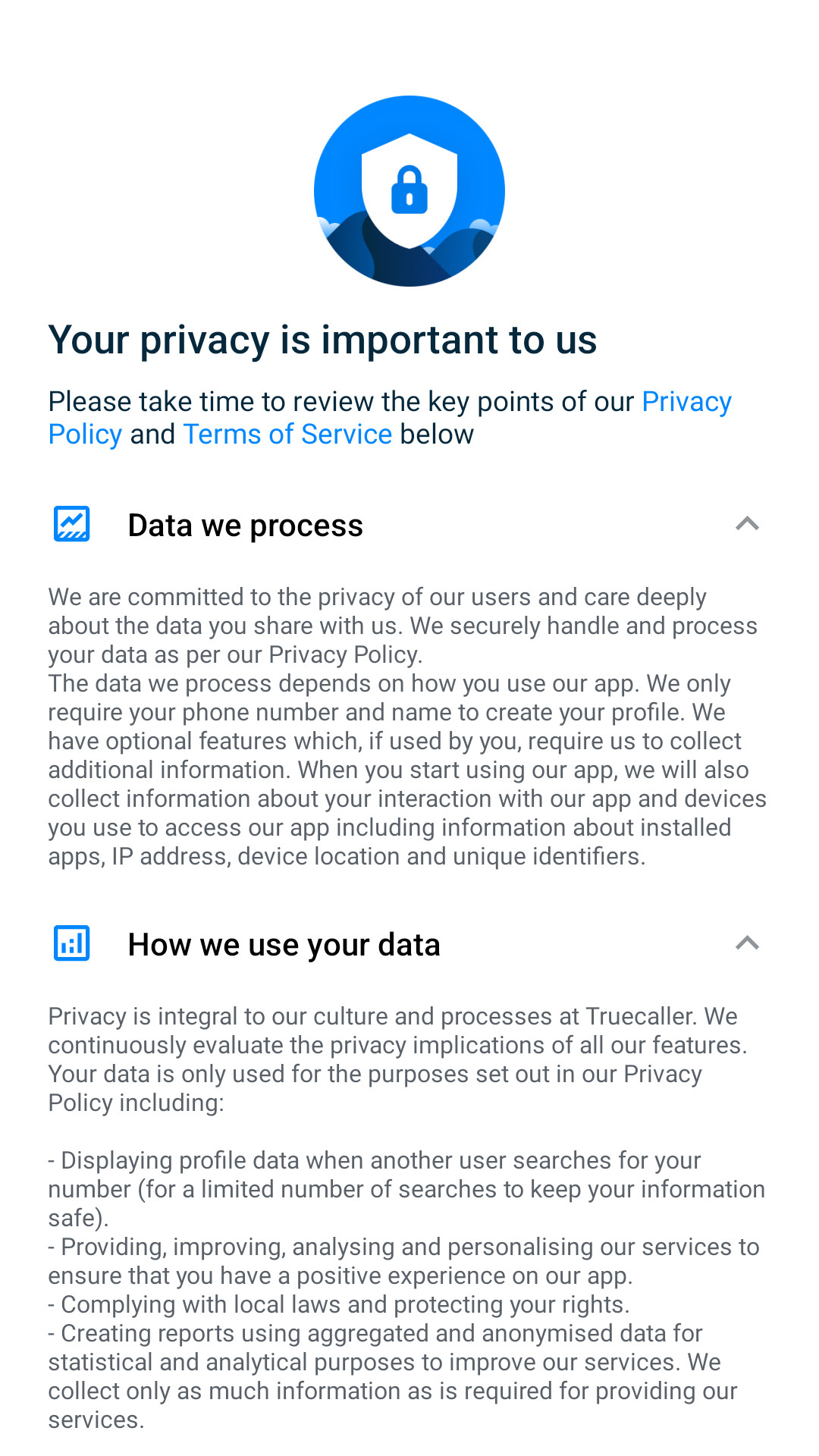In the provided image, a prominent circular emblem showcases a detailed design featuring three-quarters filled with a striking blue to represent a mountainous landscape, topped with a couple of mountaintops. At the center of this emblem is a white shield adorned with a secure blue lock symbol, signifying protection and trust. Beneath this emblem, a clear and concise message in black lettering reads: "Your privacy is important to us. Please take time to review the key points of our privacy policy and terms of service below." Both "privacy policy" and "terms of service" are highlighted in blue, indicating clickable or significant terms.

Accompanying this central message are two informative icons. The first icon, a square with a trajectory graph, is labeled "Data We Process." It explains that the company is deeply committed to user privacy, securely handling and processing user data in alignment with their policy. The second icon is a small square depicting a bar graph, titled "How We Use Your Data," which elaborates on the company’s dedication to privacy, emphasizing that data usage is strictly limited to the purposes outlined in their privacy policy. This comprehensive description assures users of Truecaller’s diligent privacy practices and their earnest commitment to protecting user information.